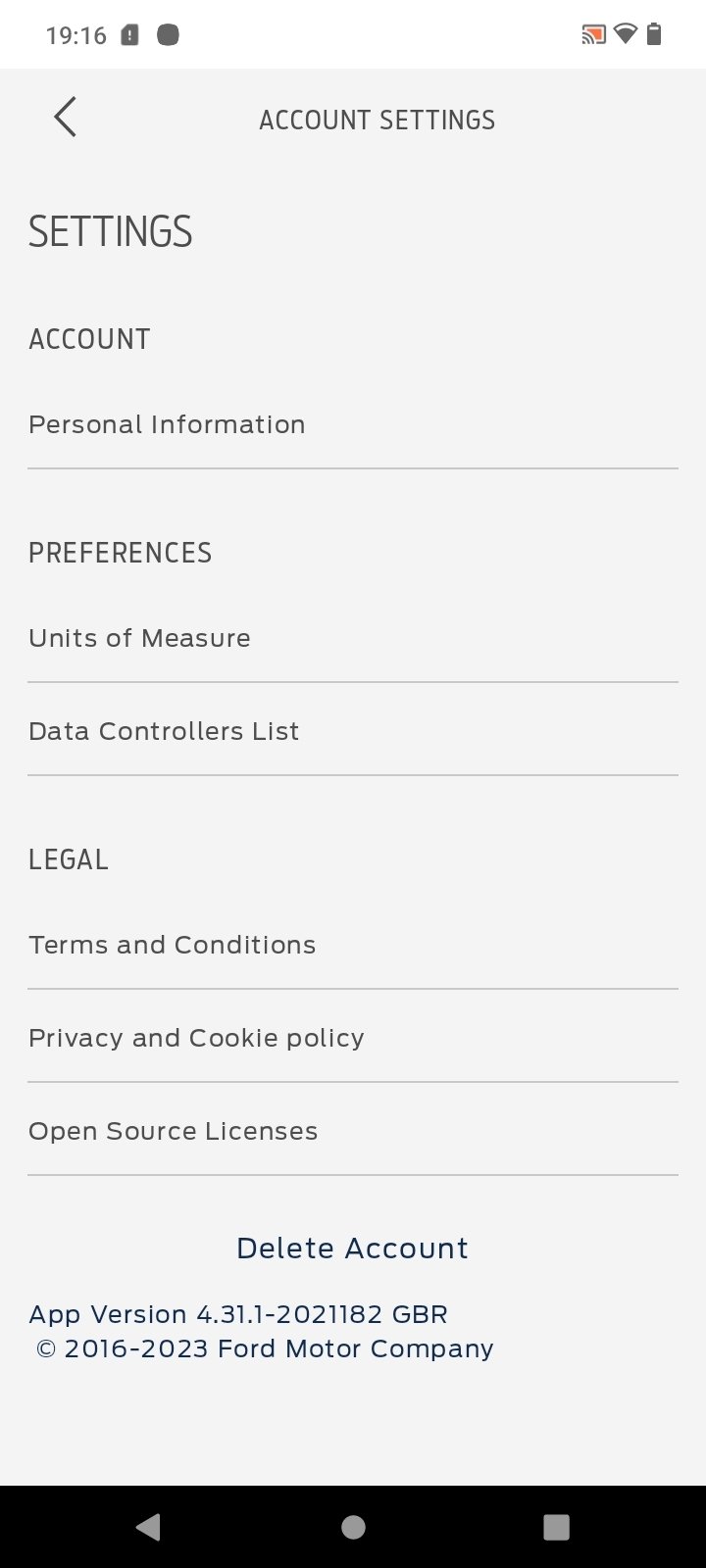The image is a detailed screenshot of a mobile device's screen taken at 19:16 (military time). The Wi-Fi signal strength is displayed with three bars, indicating a strong connection, and the battery icon shows a high level of charge. On the screen, there is a prominent header titled "Account Settings" in bold black text. Under this header, the section labeled "Account" includes "Personal Information." Below "Settings," a gray divider bar separates it from the "Preferences" section, which lists "Units of Measure," "Data," and "Controllers List." Further down, another divider bar demarcates the "Legal" section, which contains links to "Terms and Conditions," "Privacy and Cookie Policy," and "Open Source Licenses." At the very bottom, an option to "Delete Account" is displayed in blue font. The app version is specified as 4.31.1-2021182 GBR, and it is copyrighted by Ford Motor Company from 2016 to 2023. The bottom of the screen features a black navigation bar with three buttons: a back arrow, a circle (home), and a square (stop).